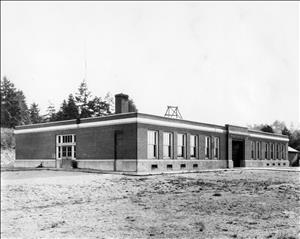This small, black and white photograph, measuring approximately two inches wide by one and a half inches high, depicts a single-story, rectangular building that appears to be of a commercial nature. Captured from an angled perspective, the image shows both the front and side of the structure. The building's façade features numerous large windows, with six visible on the right side leading up to an arched opening, with possibly six more windows beyond it. A set of double doors with windows above is located on the left-hand side, and a chimney is positioned slightly off-center on the flat roof. The ground in front of the building, which slopes gently towards the viewer, is unclear due to the grayscale tones, making it difficult to discern whether it is covered in grass or simply dirt. Framing the lower third of the image, the ground appears gray with darker spots. Towards the back left, several tall trees are visible against a washed-out gray sky. There are no identifying marks, logos, or text on the image to indicate the date or location. The photograph itself is bordered by a thin black pinstripe, enhancing its rectangular shape.